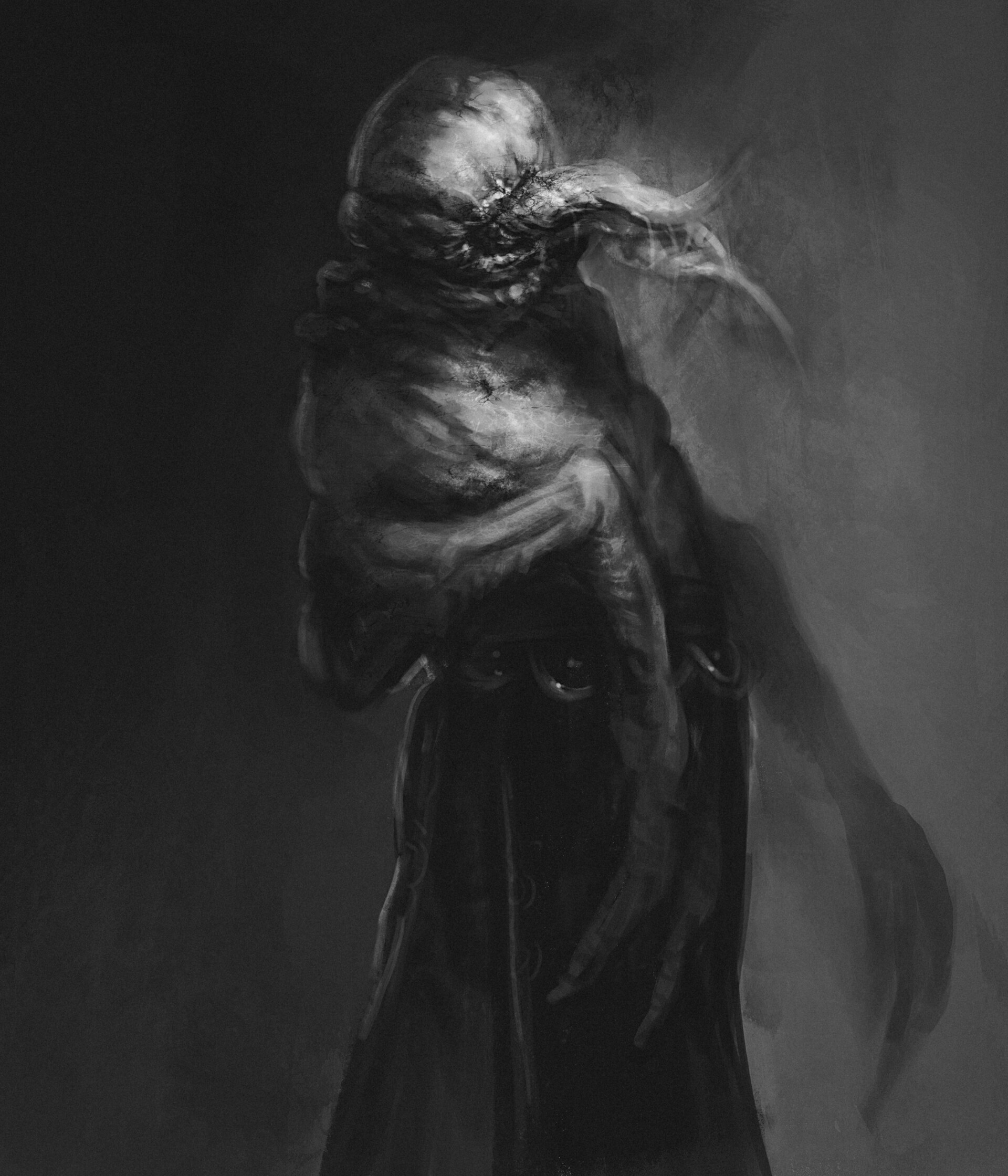This surreal and nightmarish painting portrays a malformed, humanoid horror creature set against a nondescript gray and black background. The creature appears to be dressed in a dark, black robe, although its torso is lumpy and lacks a definitive shape, combining a sense of both fatness and strength. Its arms are grotesquely deformed, transitioning from human-like upper regions to elongated claws that extend longer than its forearms. The head is devoid of eyes, featuring only a mouth from which multiple long, tentacle-like tongues emerge, possibly used as sensory feelers. This unsettling figure casts an eerie shadow on the wall, emphasizing its twisted form and adding to the overall dark and abstract mood of the painting.